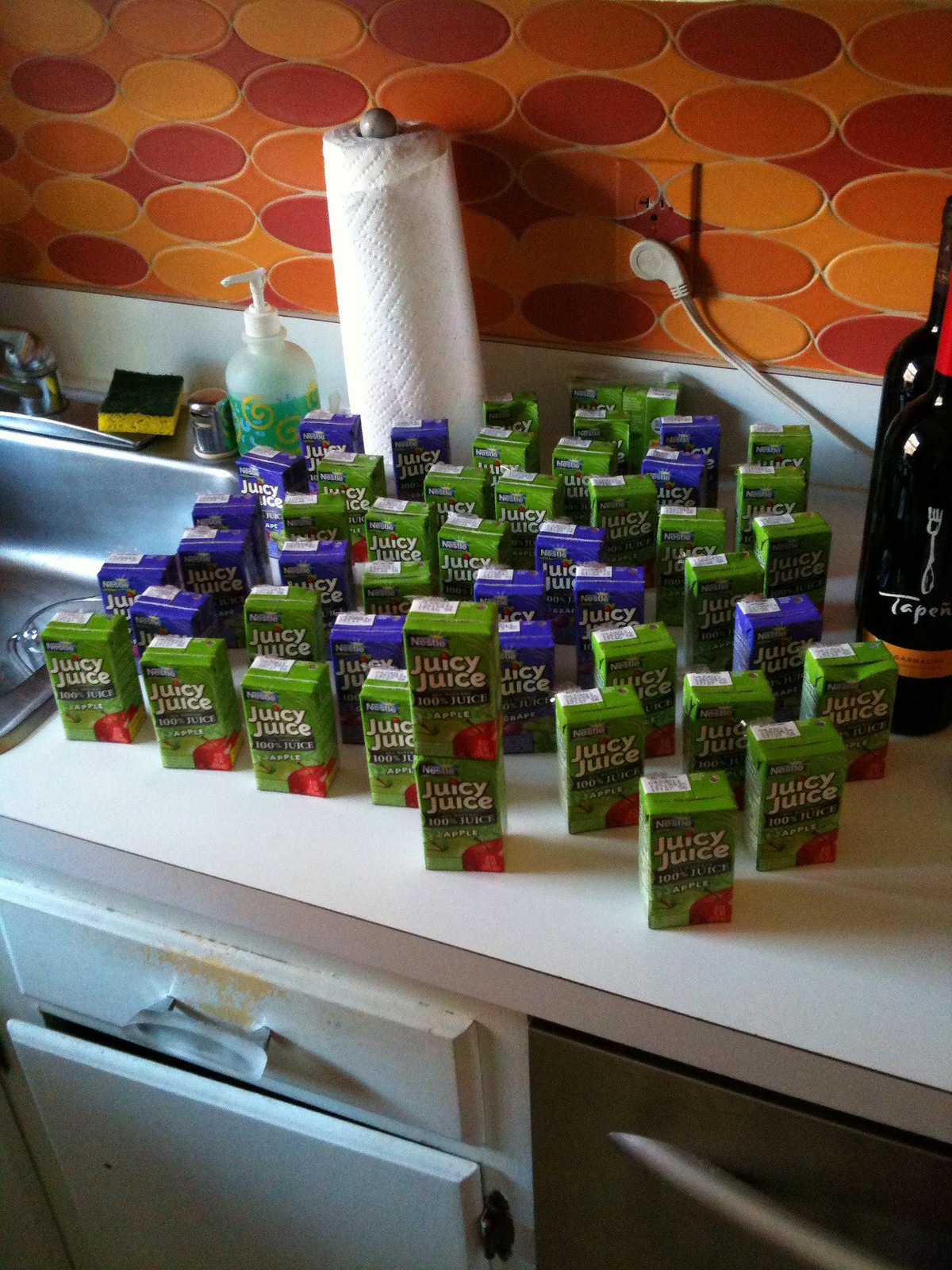The image depicts a kitchen counter showcasing a nostalgic 70s decor with a flat, white linoleum surface and slightly dingy white cabinets featuring clear plastic hardware. Central to the image is a variety of approximately 25 Juicy Juice cartons, predominantly green with an apple icon indicating 100% apple juice, alongside some blue cartons. They are positioned next to a stainless steel sink, which also houses a yellow sponge with a green scrubbing surface, a clear soap dispenser with green soap and a gold design, and a wooden paper towel holder. The backdrop consists of orange wallpaper with red ovals, giving a retro vibe. Additional items include two black bottles labeled with partially visible white lettering next to the Juicy Juice cartons, and a plug inserted into an outlet embedded in the same orange wallpaper. This kitchen image captures both a touch of modernity with functional items and a charming retro atmosphere.